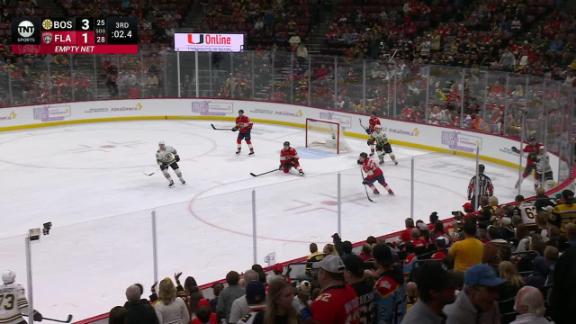The image is a landscape format, color photograph capturing a freeze frame of an ice hockey match broadcasted on the TNT television network. The scoreboard in the top left corner indicates that it is a game between Boston and Florida, with Boston leading 3-1 in the third period, and just 2.4 seconds left on the clock. The teams are distinguished by their jerseys, with Florida in red and Boston in white and black. The scene captures intense action with five Florida players guarding their empty net, as their goalie is not present, while four Boston offensive players charge towards the goal. A referee in the corner appears to be watching a potential fight between two players. The venue is filled with a large number of enthusiastic fans, who occupy about half of the visible stands, many of whom are standing and raising their hands in excitement. The perimeter of the rink is enclosed with plastic barriers, standard for hockey arenas.